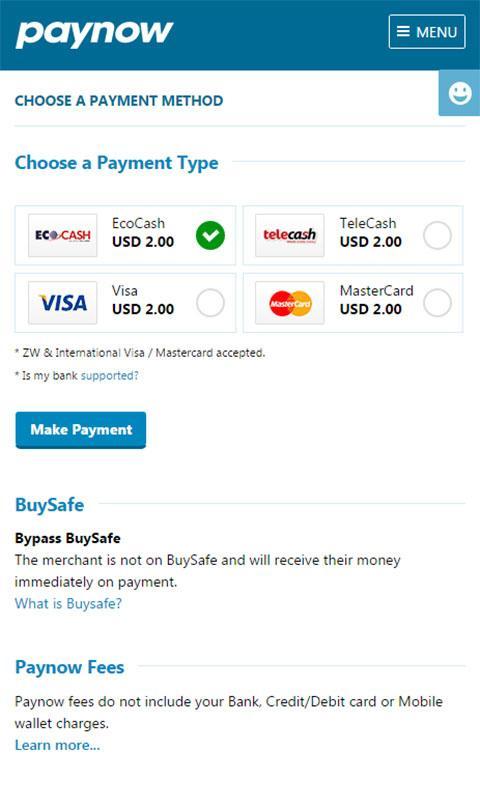In the image, there is a screenshot of a payment app called PayNow. The PayNow logo, presented in white stylized text, is prominently displayed on a blue banner at the top left corner. To the right, there is a menu button with a hammer symbol next to it. Below this, in blue text, it reads "Choose a Payment Method," next to a smiley face icon with an open mouth, which has a white face. Directly beneath the smiley face icon, it says, "Choose a Payment Type." 

The app offers four distinct payment types, each accompanied by a small circle for selection, which can be marked with a green checkmark. The selected payment type in the screenshot is EcoCash, positioned at the top left. The other available options are Visa on the bottom left, Telecash on the top right, and MasterCard on the bottom right. Each payment type corresponds to a USD amount of $2.

At the bottom of the payment options, there is a blue "Make a Payment" button with white text. Below this button, there is additional information indicating "Buy Safe" and mentioning "Bypass Buy Safe." Just below this, it references "PayNow Fees," suggesting there may be additional fees associated with using the PayNow service.